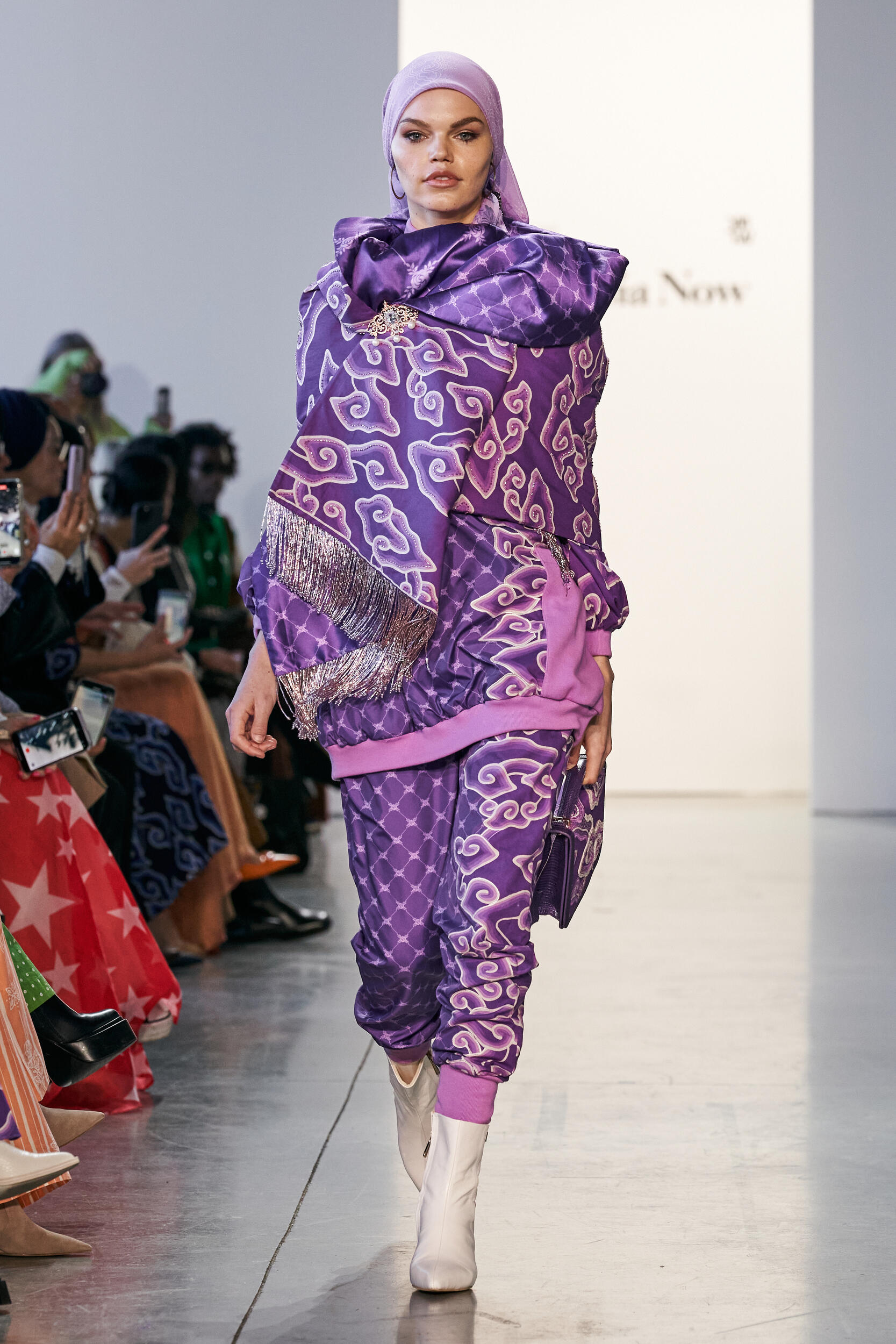In this striking photograph taken indoors, a poised model struts confidently down a runway, surrounded by a captivated audience seated to her left, their cameras and phones aimed eagerly in her direction. She sports an eye-catching, coordinated ensemble that includes white boots and vibrant purple pants adorned with a cloud-like pattern, ending in distinct cuffs just below her knee and perfectly paired with her boots. Her long-sleeved top, matching her pants, features a purple edge and is complemented by a thick, flowing purple scarf draped elegantly around her neck. A matching handbag dangles from her left arm. Adding to her stylish look, she wears a light purple head wrap, neatly tied in place. Her makeup is subtle, accentuating her natural beauty. Illuminated from behind, she casts a shadow across the runway floor, stepping out from an area with text partially obscured by her figure, save for a blurry "NOW." The overall scene radiates an air of sophistication and composure, with the model commanding the runway effortlessly in her bold, geometric-patterned, and satiny-textured outfit.